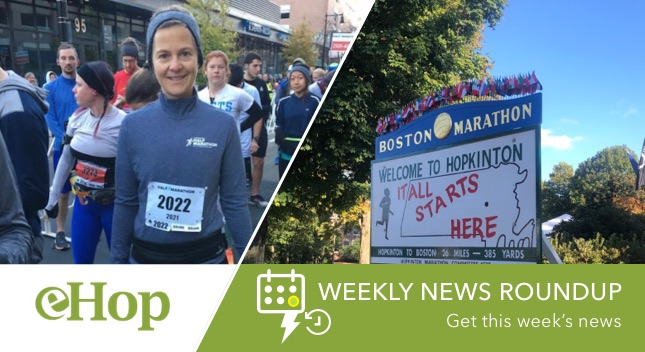The advertisement titled "eHop" is a wide rectangular image featuring a vibrant outdoor scene, split diagonally into two distinct sections. On the left side, there's a photograph of marathon participants, with a Caucasian male runner wearing a blue hat and blue running jersey prominently in the foreground, smiling at the camera with the number 2022 on his jersey. Surrounding him are several other runners, some wearing race tags, in what appears to be a bustling pre-race atmosphere, with shops and a clear sky visible in the background. On the right side, there's a sign that reads "Boston Marathon. Welcome to Hopkinton. It all starts here," overlaid on an outline of the state of Massachusetts, with a silhouette of a runner included in the design. At the bottom of the advertisement, the text "eHop" is displayed in green font on a white background on the left, while the words "Weekly News Roundup" appear in white font on a green background on the right. There are also small icons, possibly a calendar with a lightning bolt and a clock with a pointer, adding further visual elements to the lower part of the ad.